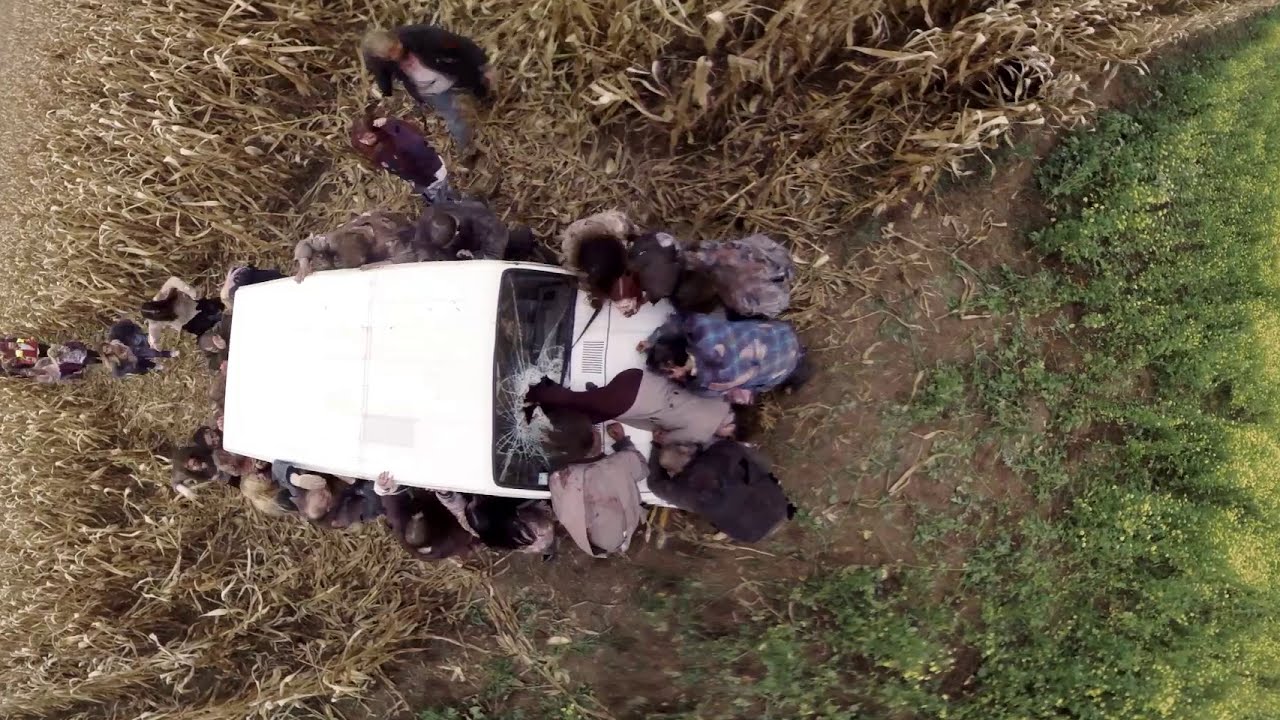In the center of a cornfield, a white box-shaped van with a smashed windshield sits amidst the golden-brown cornstalks. The impact suggests a violent crash, and a man lies injured on the hood, his legs still entangled in the broken glass. Around 20 individuals, including some appearing bloodied, surround the vehicle, particularly focusing on the injured man at the front. The scene, captured from an overhead perspective with a slight fisheye lens effect, emphasizes the chaos and urgency, resembling a dramatic movie still. The setting is rural, likely a farm, with some grass visible to the right side, differentiated by varying shades of green, yellow, brown, and flecks of purple, pink, and blue scattered among the crowd. This image, stark and gripping, is devoid of any text, placing the entire focus on the surreal and haunting tableau it presents.